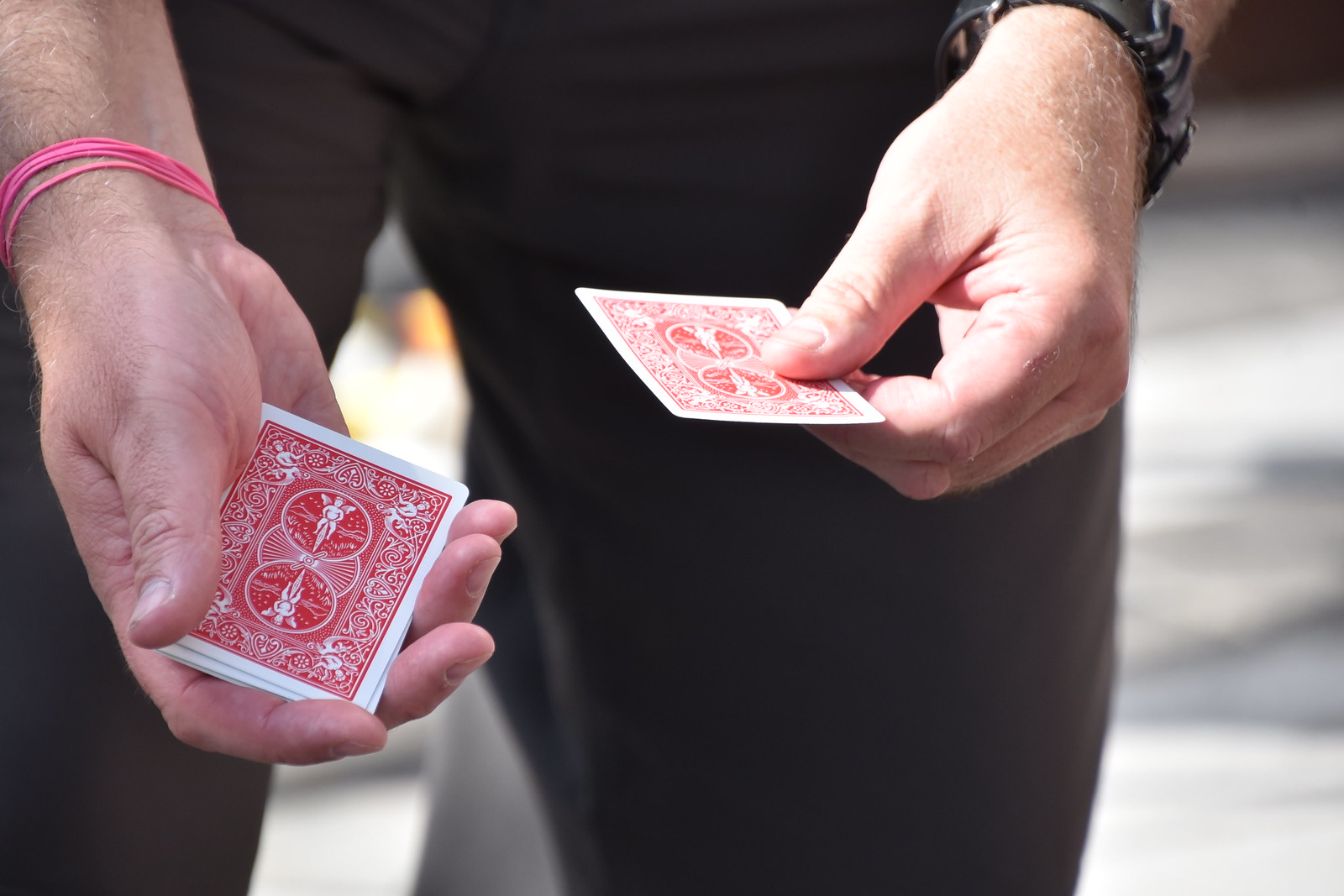In the image, two hands are prominently featured holding playing cards against a white background. The hands appear to be male, although this isn't certain. The individual is dressed in black pants, with the frame capturing from the upper part of the legs down to just above the knees. The right hand, which is positioned on the left side of the image from the viewer's perspective, holds a single card horizontally. This hand is adorned with a black leather bracelet accentuated by metallic elements, suggesting a fashionable accessory rather than a traditional watch. The left hand, conversely, is embellished with four pink elastic bands and holds a small stack of cards, approximately three or four, that are oriented towards the photographer. The background remains largely unadorned, emphasizing the focus on the hands and the playing cards with their distinct red designs.